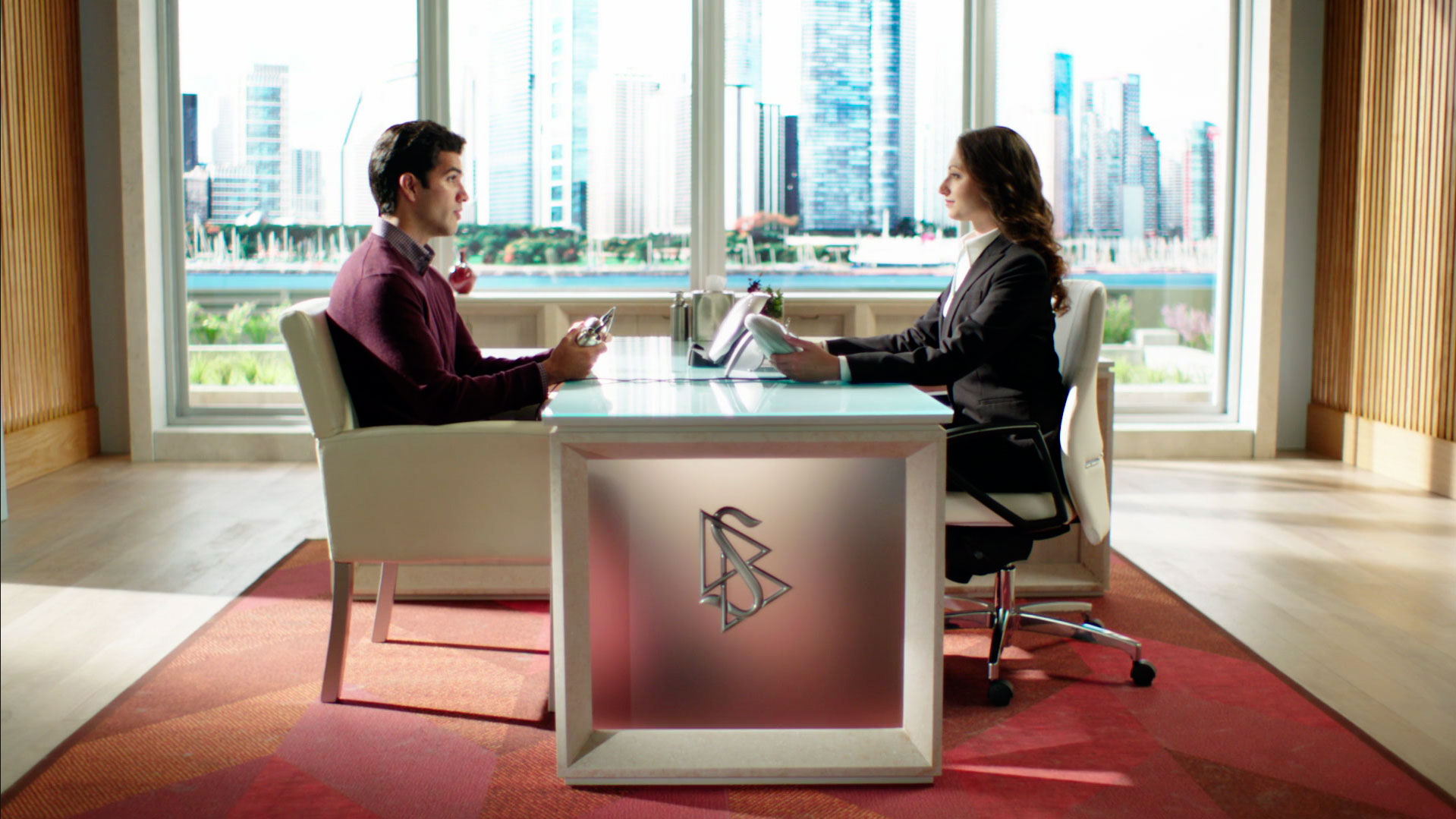In a spacious office setting, two individuals sit across from each other at a central white desk adorned with a distinctive "S" logo and two triangles. The woman, dressed in a dark-colored business suit, sits to the right in a white wheeled office chair, while the man, wearing a maroon sweater over a collared shirt, occupies a stationary white chair on the left. Beneath them lies a rectangular, multi-hued area rug featuring shades of red, orange, and pink. The room is characterized by floor-to-ceiling windows with wooden frames, providing a view of a cityscape outside. Vertical wood paneling flanks the windows on either side. A computer rests on the desk, and the two individuals engage in an intense, focused exchange.